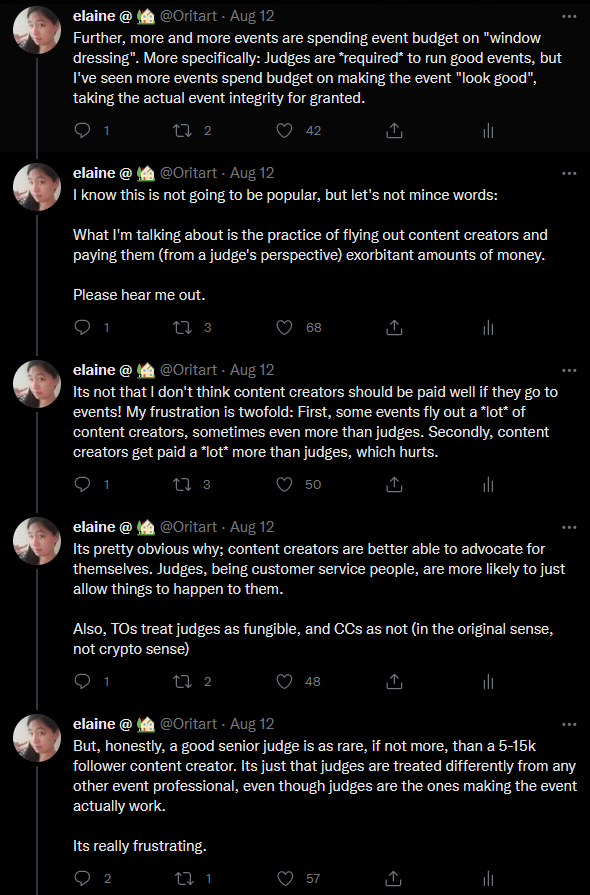This image displays a social media post featuring a dark background. Central to the image is a photograph of a woman named Elaine, accompanied by text that discusses an issue within the events industry. The text reads:

"Elaine - August 12th

It's concerning how some events allocate their budgets on superficial 'window dressing' rather than ensuring the integrity of the event. More specifically, 'judges are required to run good events,' but I've noticed a trend where more money is spent on making the event 'look good' rather than preserving its true quality. Though this opinion might not be popular, it needs to be addressed. This practice includes flying out content creators and compensating them."

The post has gathered engagement, indicated by a chat symbol, a single reshare, a heart icon with 42 likes, a share icon, and a bar graph, all showing various interactions with the post.